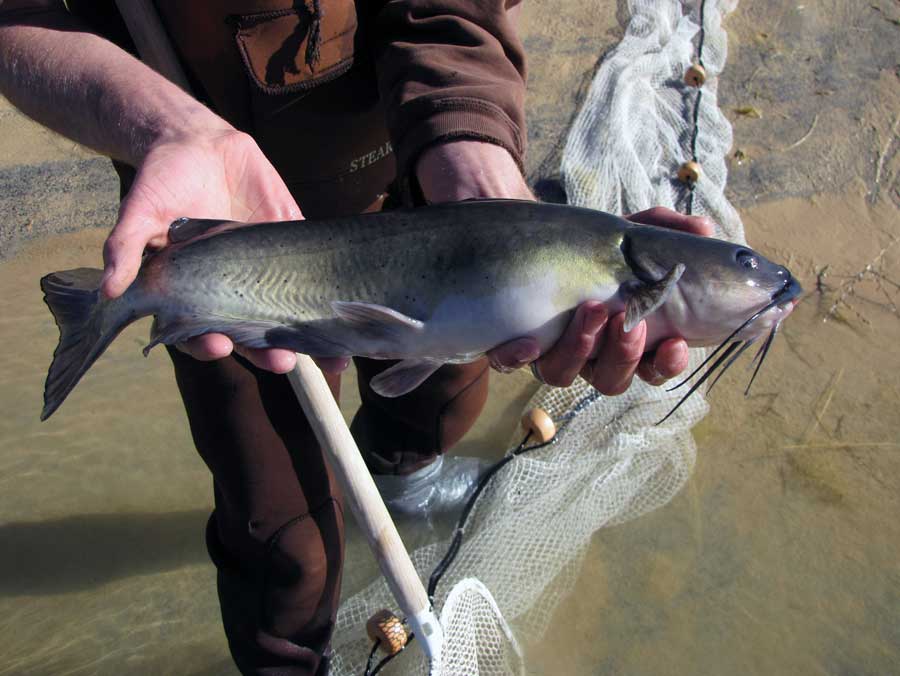This real-life photograph captures the moment a fisherman proudly displays his sizeable catch by a riverbank. The man, dressed in heavy-duty brown coveralls and a matching long-sleeve sweatshirt, holds a large catfish with distinctive long black whiskers. His outstretched hands cradle the fish, drawing attention to its impressive length and the contrasting colors of its body—mostly black with a white belly and a few gold and black spots. Standing in the muddy, silty waters near the shore, the man is braced against a net, which is partially submerged and also held by him. Grayish boots protect his feet as they stand amidst scattered grasses and debris, adding to the rugged, natural setting.